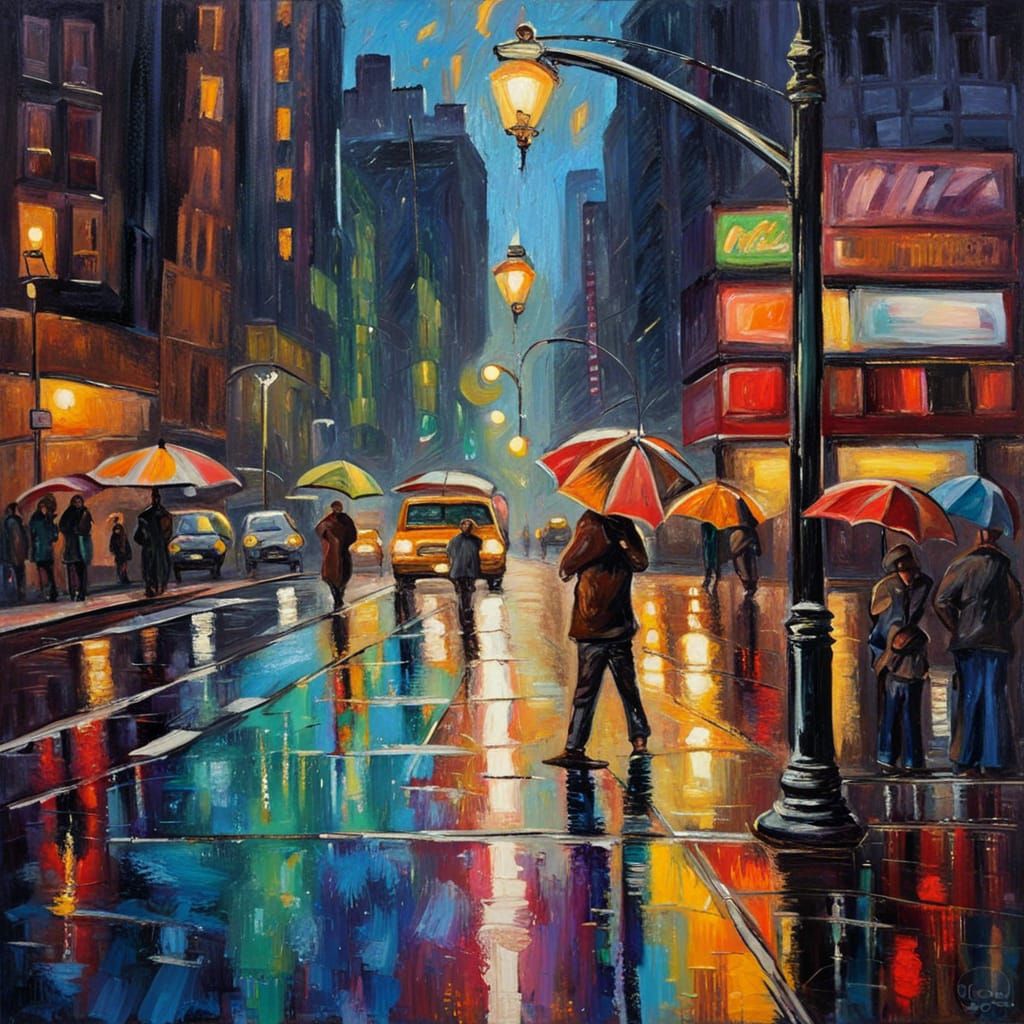This painting depicts a rainy city street scene at night, rendered in a slightly modern take on Impressionism. The street is alive with numerous pedestrians carrying umbrellas of various colors and patterns, with red and orange recurring prominently among a variety of blue, green, and yellow. The wet street reflects a kaleidoscope of vibrant lights from the surrounding environment, including street lamps that line the center of the street, receding towards the horizon. Tall buildings rise on either side, their windows and sporadic commercial signage contributing subtle glows to the atmosphere. A distinct yellow car, likely a taxi, approaches the viewer with its headlights on, while other vehicles are parked along the street. The ethereal blue sky peeks through, suggesting that dusk has fallen, but the multitude of bright colors—gold, pink, and orange—casts a lively spirit over the misty scene. The people, though numerous, blend into the background, allowing the vivid umbrellas, shimmering street reflections, and illuminated architectural details to dominate the composition.